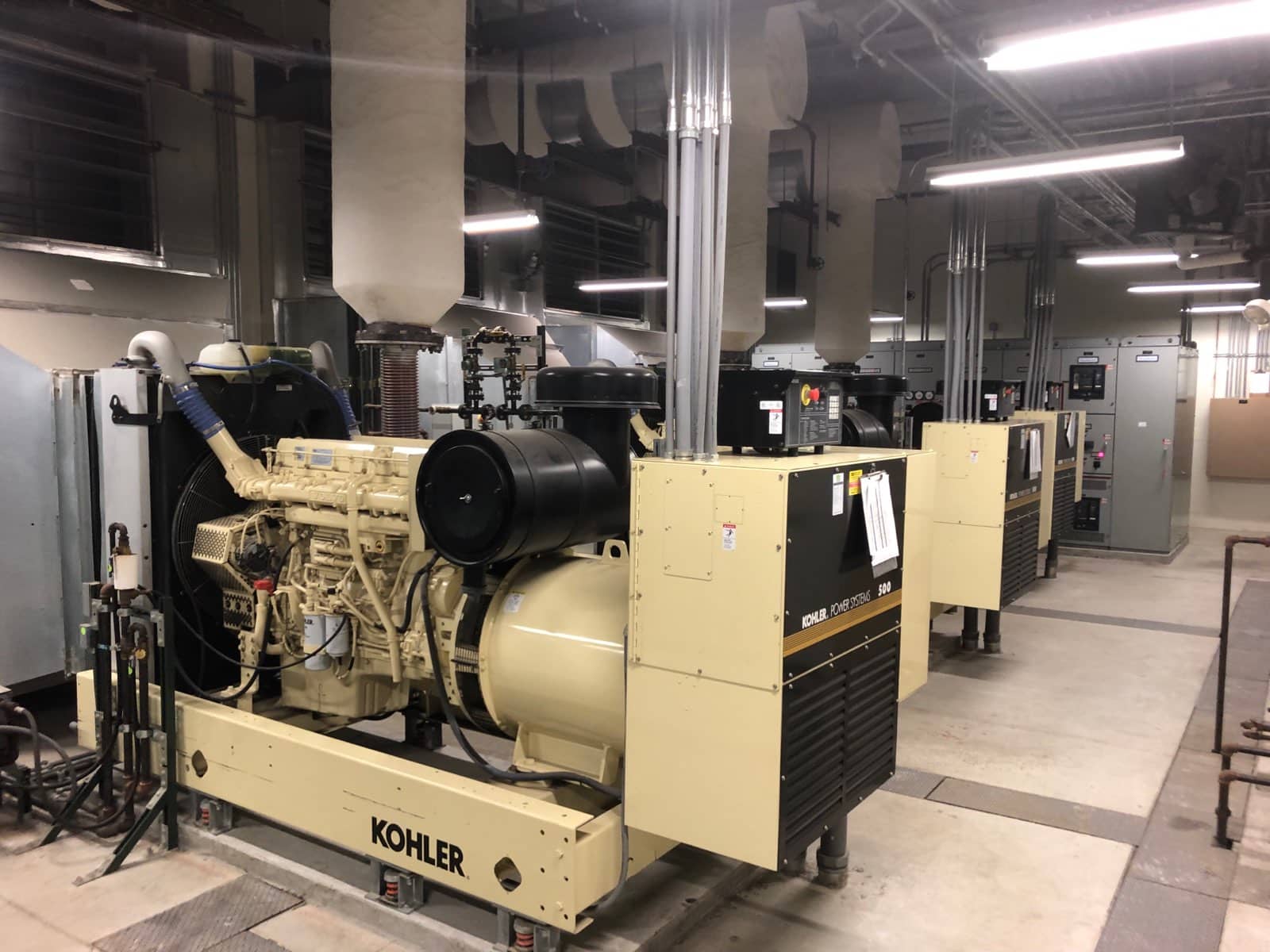The image depicts a large industrial or laboratory setting, fully illuminated by overhead fluorescent lights. Dominating the scene are three heavy-duty machines branded as Kohler Power Systems 500. Each machine features a prominent cylindrical tank connected to a pump, and above these tanks, an overhead pump interfaces with the machine's core. Tags or instructions are affixed to the front of each unit. To the right of the tanks, a box houses electrical components, and gray tubing extends upwards. The machines, which appear aged, may function as generators or compressors. In the background, security devices or lockers line the space, and there are visible pipes and mainframe circuitry, underscoring the complexity of the environment.